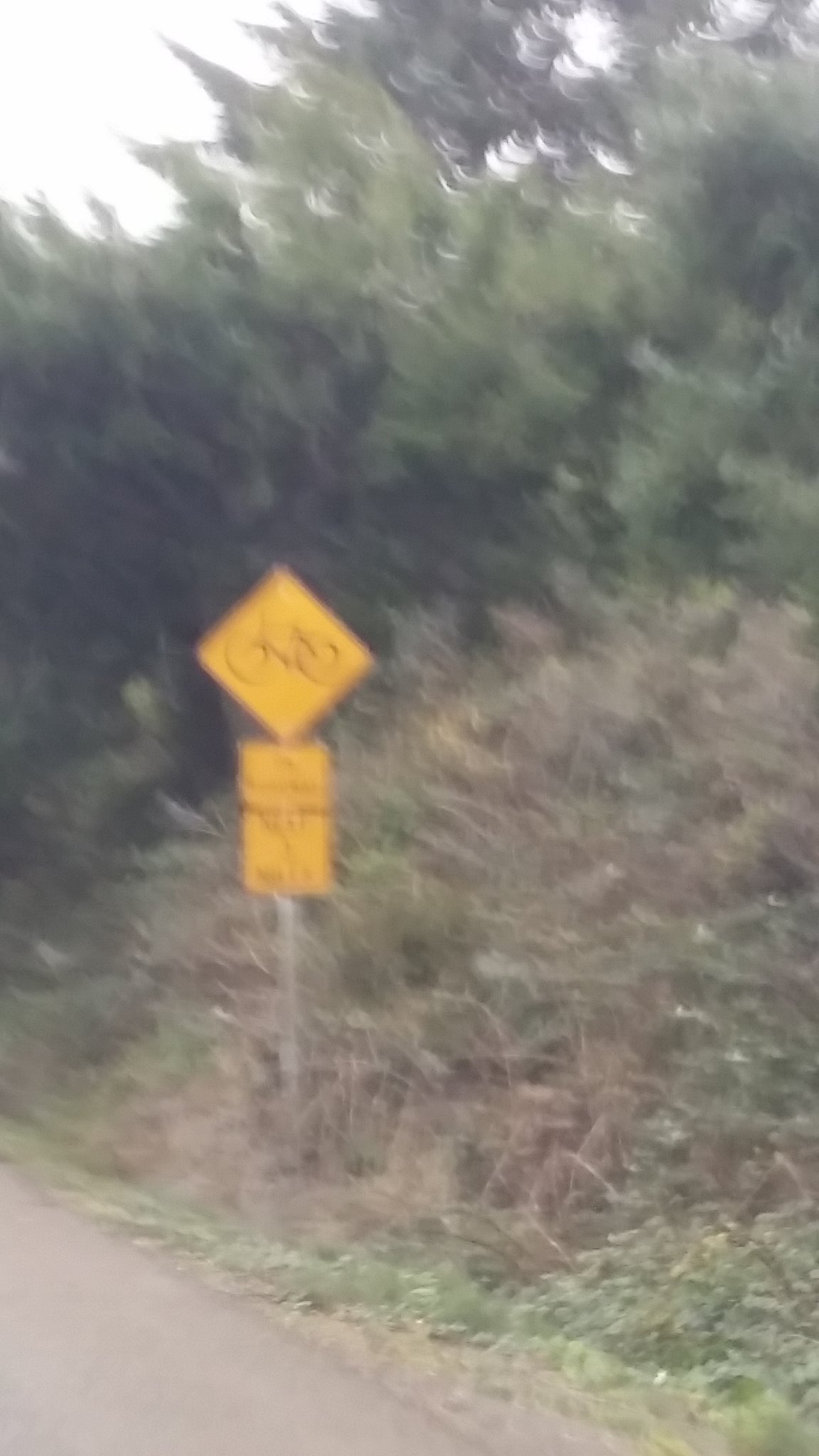In this very blurry and dimly lit image, a street sign stands amidst a mix of green and brown vegetation, suggesting an early fall scene. The sign is mounted on a wooden post and comprises three parts: the topmost is a square yellow sign with a black bicycle silhouette, below which are two rectangular signs with unreadable text due to the blur. The lower left corner of the image reveals a small section of a paved road, which then slopes steeply upward into a wooded hillside covered in grass, weeds, and a combination of green and tan foliage. The background features large bushes and a prominent evergreen tree set against a white sky.